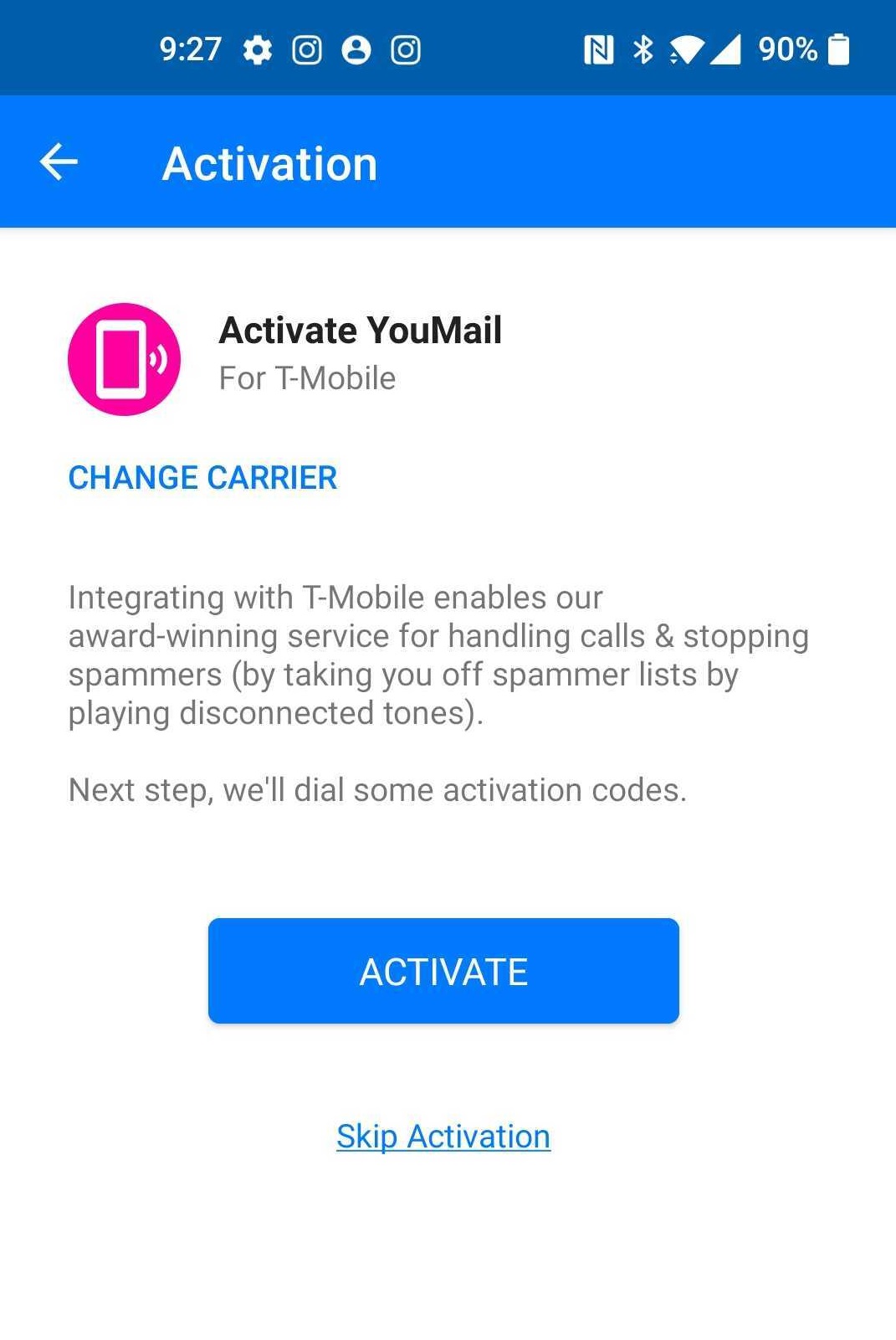The image depicts a detailed process of email activation for T-Mobile service. At the top of the screen, there is a dark blue header displaying the time as 9:27, along with several icons: settings, a profile icon, a box with an 'O' and a circle in it, and another box with a circle in it. To the right, the icons indicate a battery level at 90%, good signal strength, and active Wi-Fi.

Below this header, a lighter blue box is titled "Activation," accompanied by an arrow pointing to the left. The bulk of the screen features a white background.

On the main portion of the screen, there is a prominent pink circle containing a phone icon. Text adjacent to this reads, "Activate email for T-Mobile," with "Activate email" in black letters. Beneath, in light blue, the words "change carrier" indicate an option to switch service providers.

A detailed explanatory note in gray text states, "Integrating with T-Mobile enables our award-winning service for handling calls and stopping spammers by taking you off spammer lists by playing disconnected tunes." The next step in the process involves dialing activation codes.

Toward the bottom of the screen, a blue button labeled "Activate" prompts further action. Below this button, teal letters reading "Skip activation," underlined, offer an alternative option to proceed without activation.

This detailed layout clearly guides the user through the email activation process for T-Mobile, highlighting options for service enhancement and protection against spam.